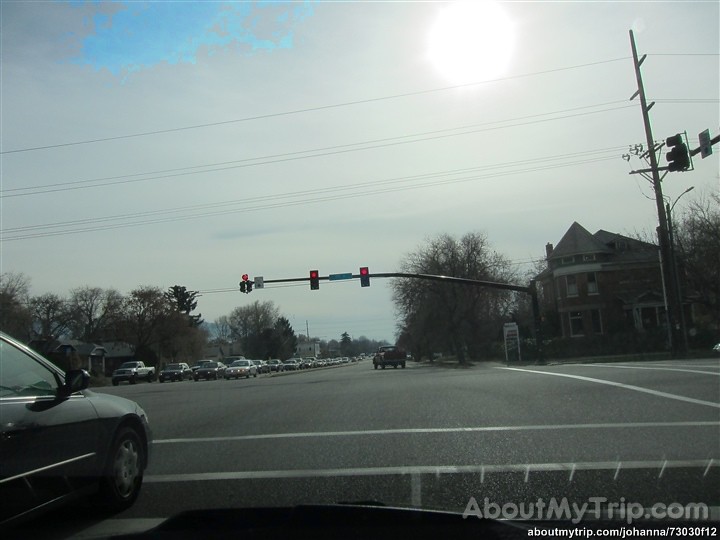The image, seemingly captured by a dash cam with the watermark "aboutmytrip.com" in the bottom right corner, depicts a four-way intersection with a road extending forward and another turning to the right. Prominently, a horizontal bar mounted on a post to the right supports three traffic lights, all currently red—two above the straight lanes and one for the left turn lane. Additionally, the post bears two signs displaying the street name and a warning. 

In the oncoming lane to the left, numerous cars are waiting at the intersection, while only a few cars are seen in the forward lane. A large house or possibly a business establishment stands on the right corner beyond the intersection, notable for its three floors, a rounded turret-like structure, and a pyramid or conical-shaped roof. In front of this house is another traffic light for the cross street, and power lines are visible overhead, crossing the intersection. Leafless trees and the setting sun in the sky suggest an autumn or winter afternoon, and the scene captures a typical moment of urban life paused at a traffic signal.